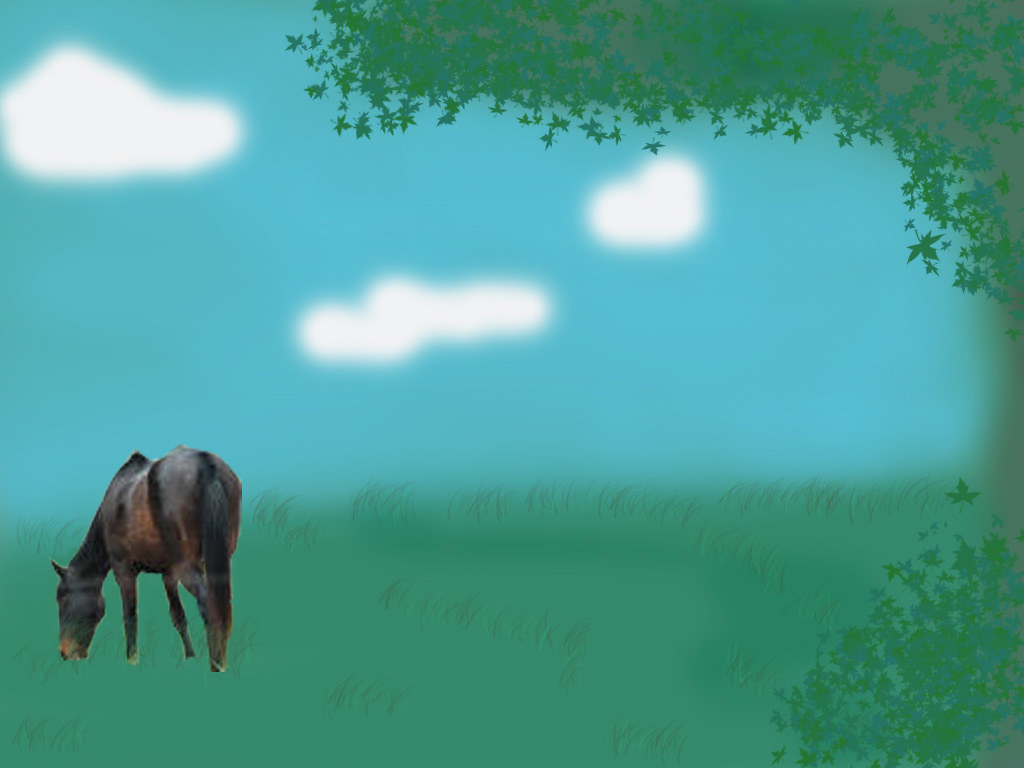The image is a computer-generated composite featuring a realistic photograph of a dark brown horse kneeling down to graze, set against a digitally created background. The backdrop portrays a grassy field with a few sparse blades of grass depicted with minimal texture, giving it a somewhat plain appearance. To the right, green leaves are clustered, suggesting the presence of a tree that extends toward the middle of the image. Above, three blurry white clouds float in a blue sky, enhancing the painted or sketched aesthetic. Despite the simplistic shading of the grass and the childlike rendering of the clouds and leaves, the scene is unified under a large tree that dominates the upper portion. The horse itself has a long black tail, and its coat appears darker with subtle lighter patches that might suggest a saddle, and it is positioned in the lower left part of the image, immersed in the grass with its face down as if munching.